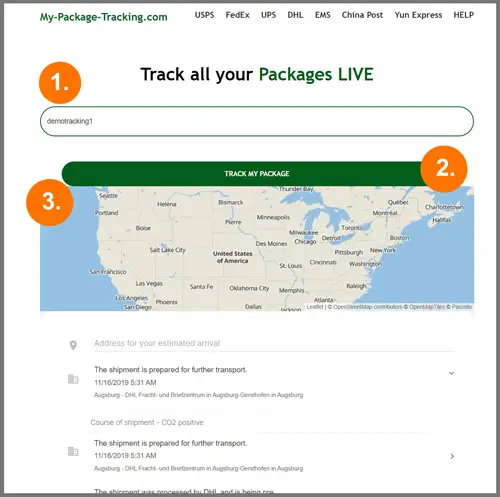**Screenshot of My-Package-Tracking.com Interface**

The image is a screenshot of the My-Package-Tracking.com website. The interface has a distinctive black border surrounding a white background. At the top-left corner, the site name "my-package-tracking.com" is prominently displayed in green. Below this, there is a navigation bar with several tabs listed in black, including options for UPS, USPS, FedEx, DHL, EMS, China Post, Unixpress, and Help.

A large, orange circle marked with the number "1" appears prominently near a wide text input field, where users can type in their tracking information. Adjacent to this field is a green button labeled "Track My Package."

To the right of this section, there is another large orange circle marked with the number "2." A third large orange circle marked with the number "3" is visible slightly lower on the left side of the interface.

In the middle section, there is a wide rectangle featuring a map of the United States, stretching from Seattle in the northwest to Dallas in the southern midsection, with the Atlantic and Pacific Oceans visible on either side. Major cities are labeled on this map.

Beneath the map, there is additional information written in black text, though it is difficult to discern due to the resolution of the screenshot.